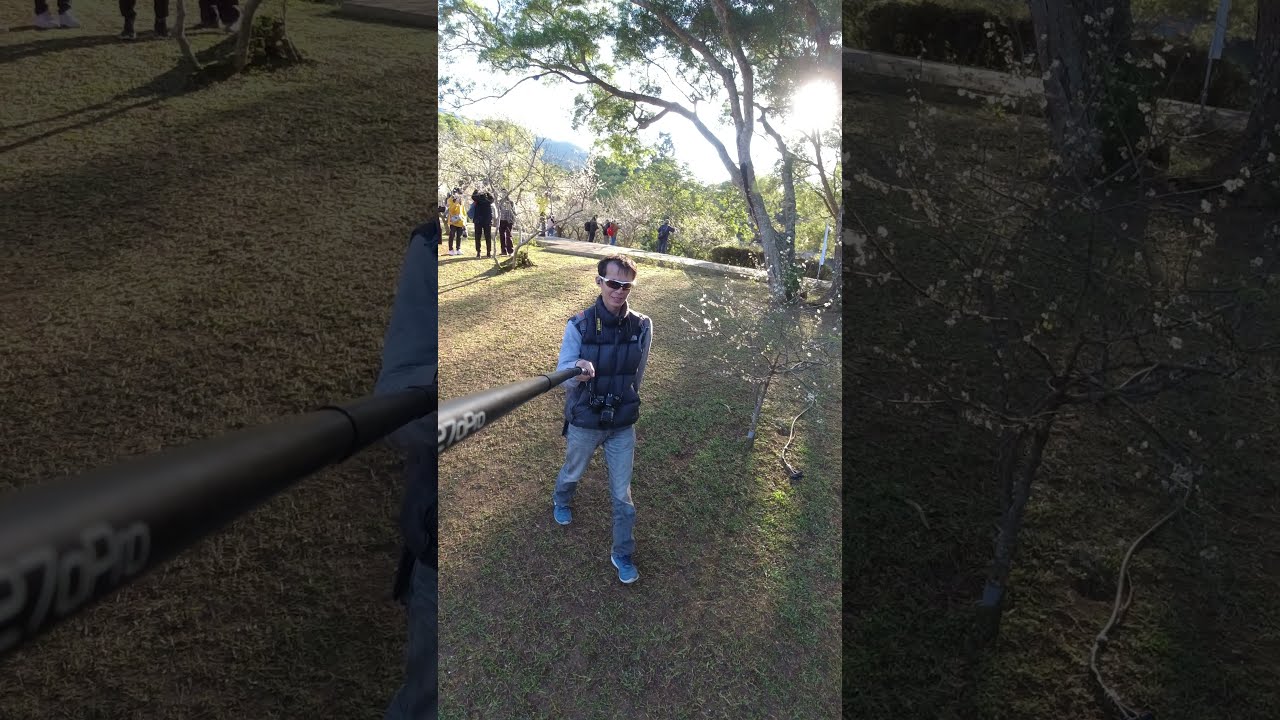A young man, possibly of Asian descent, is the central figure in this daytime outdoor photograph. He is outfitted in a dark blue utility vest over a light blue shirt, complemented by blue jeans and matching blue sneakers. His short hair is partially concealed by white sunglasses that cover his eyes. The man holds a black selfie stick in his right hand, extending slightly bent towards the camera, with the brand "270 PRO" visible on the stick. A camera with a strap hangs around his neck. He walks across a grassy field with trees in the background, where a sun flare is visible in the upper right corner of the image, suggesting a setting sun. Additional people are scattered in the top left and center of the photograph, standing on a grassy rise, watching the scene unfold. The setting appears summery with a clear blue sky overhead and mountains lining the horizon.